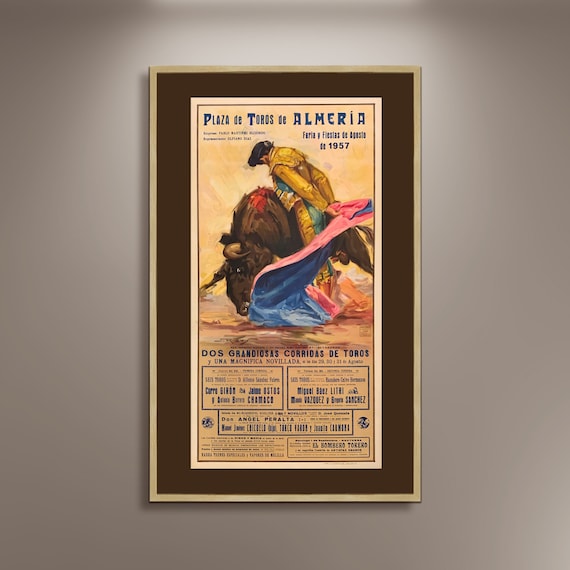In this square image, the background is a light taupe wall with a shadow or glare of white light visible at the top, possibly from the sun or an indoor light. At the center of the wall, there's a vertical rectangular poster with a gold frame and a thick brown border around it. The poster features Spanish text that reads "Plaza de Toros de Almeria" at the top in blue letters, followed by smaller, mostly unreadable print, and "Faria y Fiestas de Agosto, 1957". Near the bottom, clearer text states "Dos Grandes Corridas de Toros".

Dominating the middle of the poster is a painted graphic of a man, possibly a matador, dressed in a detailed mustard or gold and green outfit, and wearing a black hat. He is positioned in front of a brown bull, which carries a notable red mark or slit on its back. The matador appears to be holding a bi-colored cape, pink on one side and blue on the other. The artistic style of the image gives a vintage look, consistent with the poster's 1957 date.